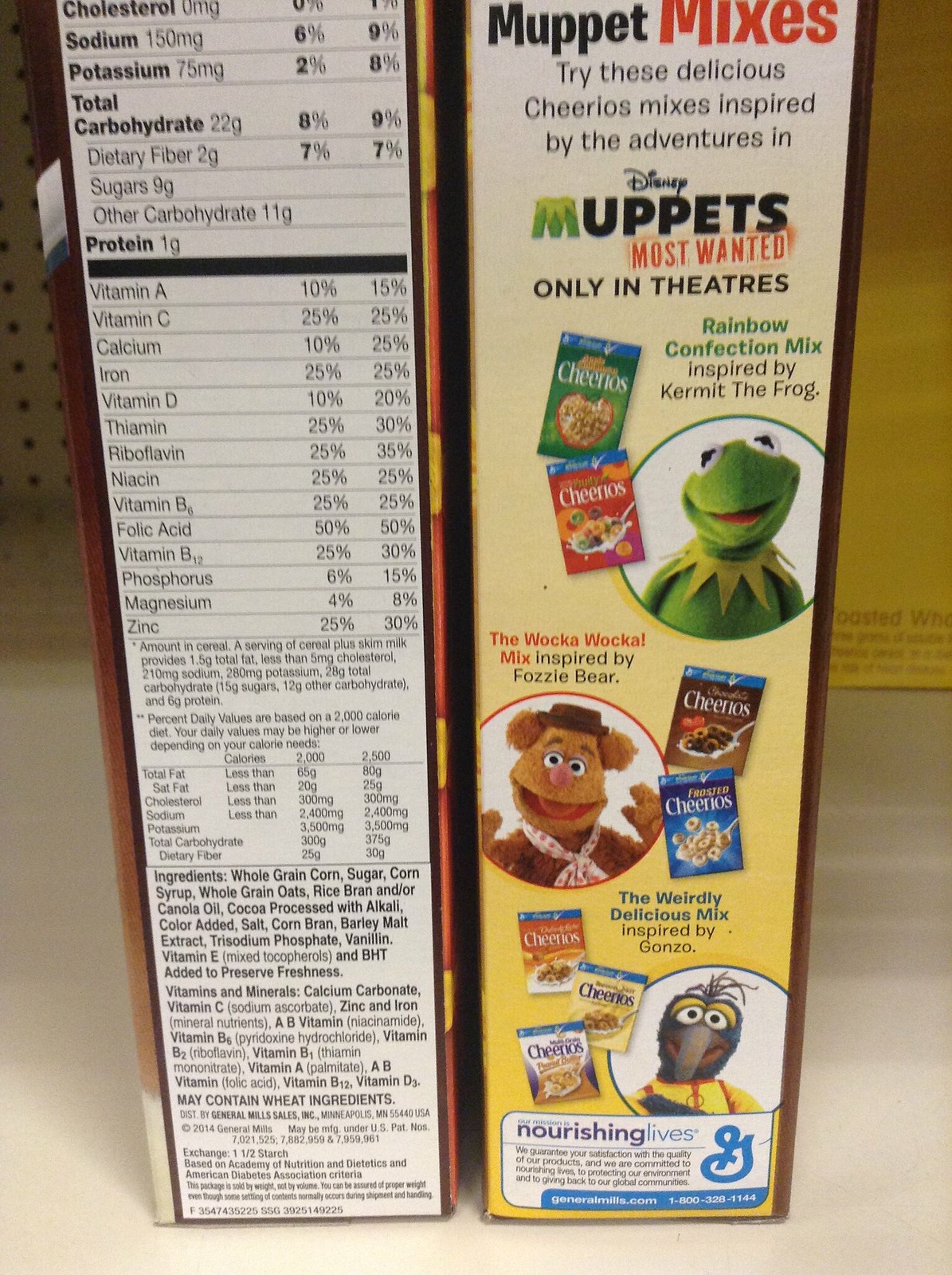Close-up view of the side panels of two cereal boxes. The box on the right is unmistakably a box of Cheerios. Prominently displayed on it is an advertisement for "Muppet Mixes," enticing breakfast enthusiasts to try delicious Cheerios mixes inspired by the Disney movie "Muppets Most Wanted," which is currently in theaters. This side panel features a vibrant image of beloved Muppet characters Kermit, Fozzie Bear, and Gonzo alongside an assortment of Cheerios varieties.

The box on the left remains ambiguous but shares similar packaging attributes, hinting it could also be a Cheerios box. It sports a predominantly yellow and orange color scheme, reinforcing this possibility. This side panel is packed with nutritional details, meticulously breaking down values for cholesterol, sodium, potassium, total carbohydrates, and proteins contained in the cereal. The overall scene captures the informative and playful juxtaposition typical in cereal box designs, blending crucial nutritional information with engaging promotional content.